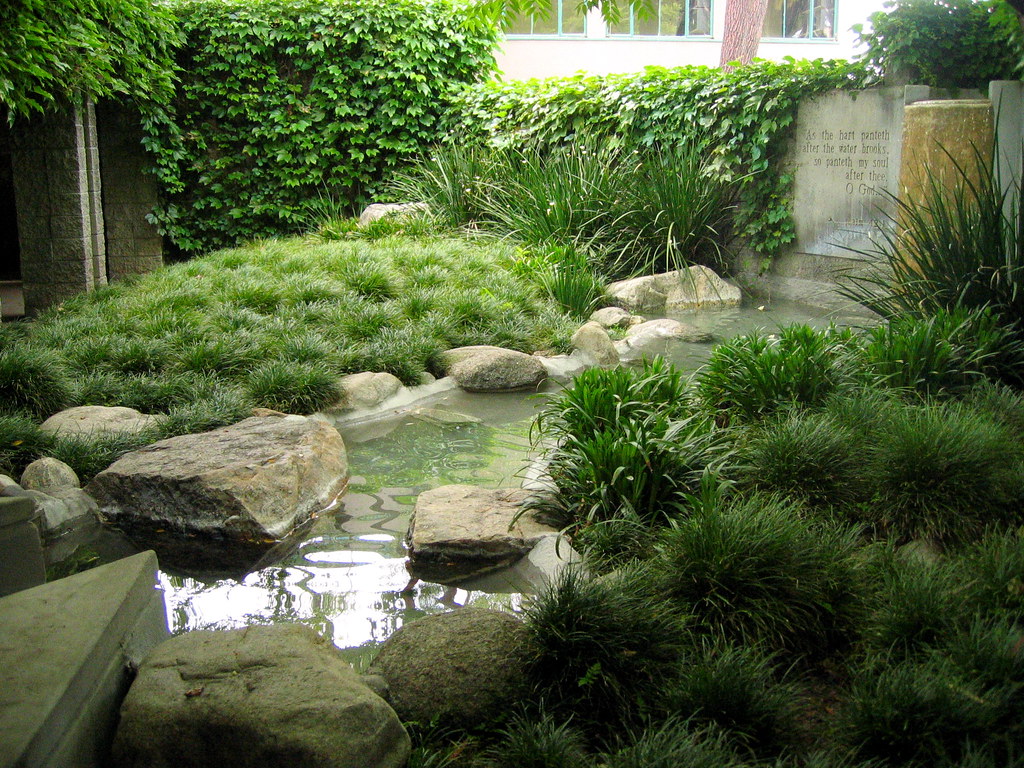This outdoor photograph, taken during daylight, showcases a serene garden setting centered around a small stream that weaves through an array of large rocks. The stream passes beneath two rectangular concrete slabs, and on both sides, lush green grass dominates the scene, particularly thick in the bottom-right corner. The top-right corner reveals a mural on a concrete wall, with a sculpted quote reading, "As the heart panteth after the water brooks so panteth my soul after thee, O God." Below the text, a series of climbing vines ascend the wall, extending over stone pillars that are adjacent to a white building partially visible in the center background. To the left of the stream, additional greenery includes grass, a few trees, and some bushes, while ornamental grasses suggest a well-cultivated garden ambience. The overall aesthetic resembles a tranquil Japanese garden, complete with a blend of natural and structured elements.